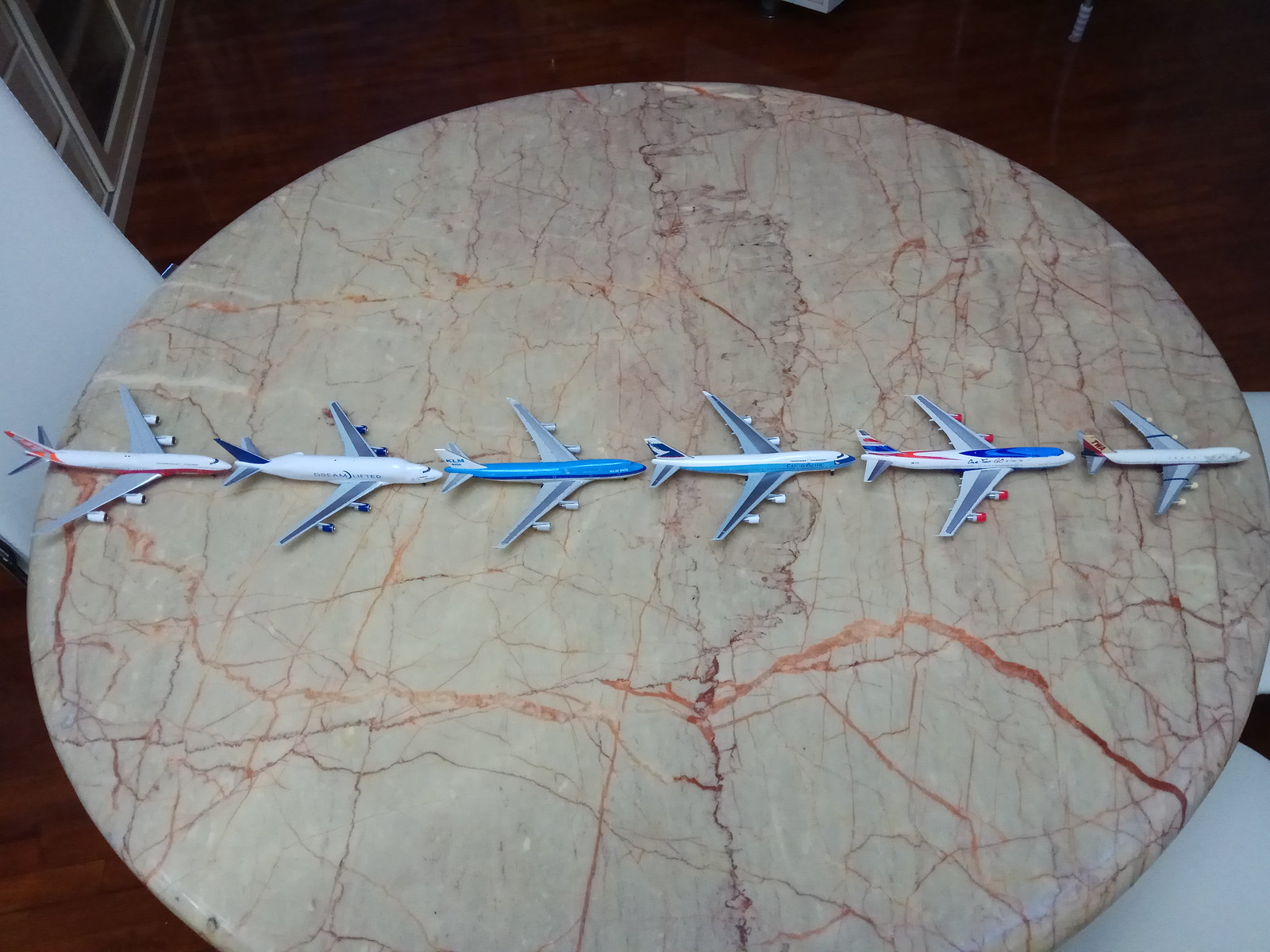The image captures a round marble coffee table inside a house, featuring intricate veining in shades of brown, red, and orange, giving it a map-like appearance. The table's surface showcases six toy airplanes, meticulously lined up from smallest to largest, each resting on their wheels. These toy planes, representing different airlines, predominantly feature white, blue, and touches of red. Surrounding the table, the wooden floor is visible, characterized by its rich brown hue. Additionally, the background includes a sliding glass door and a white pillar, adding depth to the setting.